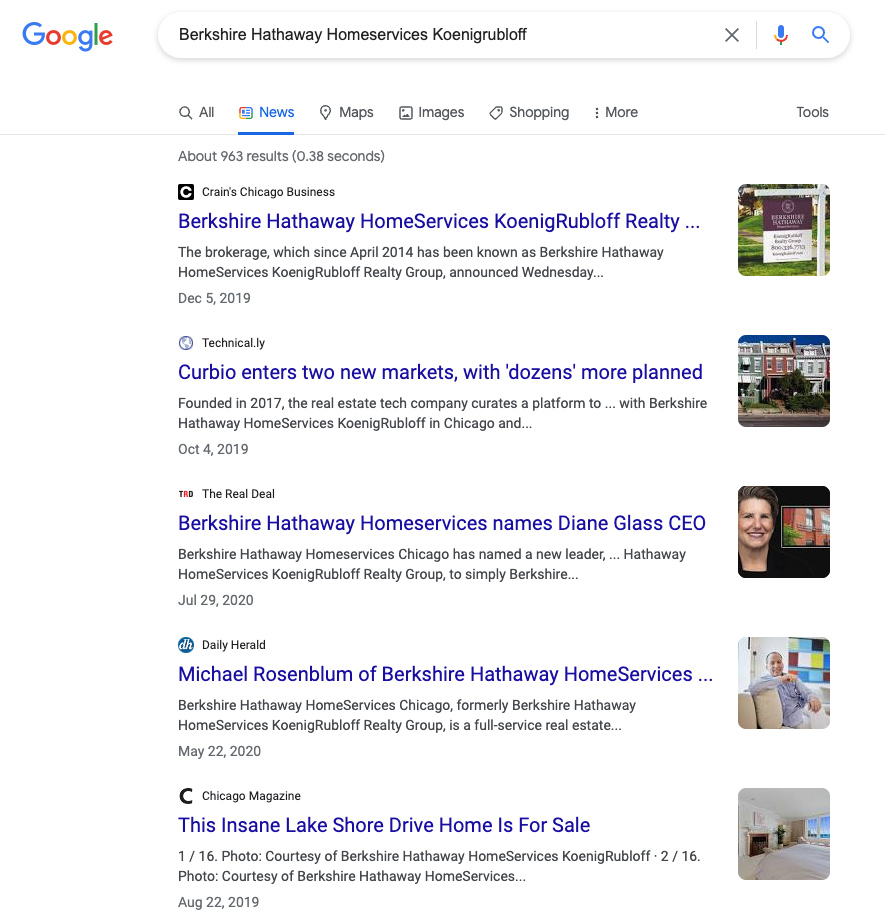A screenshot revealing Google search results is displayed. In the upper left-hand corner, the Google logo is prominently visible beside the search bar, which contains the query "Berkshire Hathaway HomeServices KoenigRubloff." Directly beneath the search bar, the navigation tabs for "All," "News," "Maps," "Images," "Shopping," and "More" are neatly aligned, with the "Tools" tab situated to the far right on the same line. Just below these options, the search results summary indicates approximately 963 results found in 38 seconds. The topmost search result leads to Crain's Chicago Business, featuring a link that reads "Berkshire Hathaway HomeServices KoenigRubloff Realty."